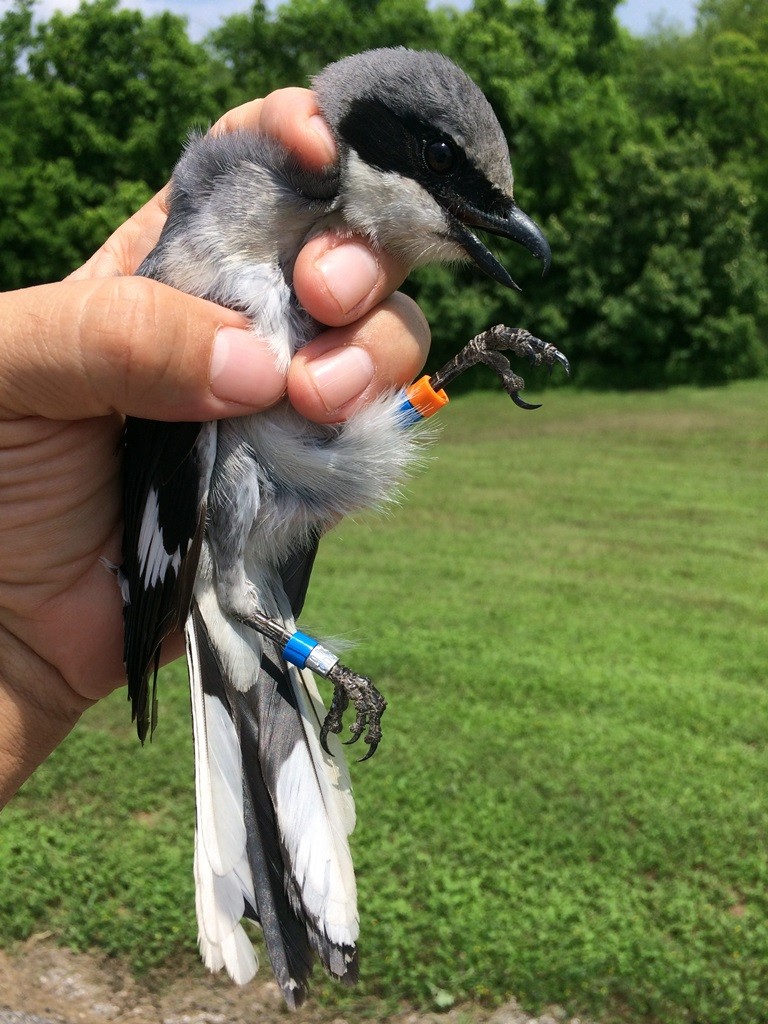The photograph captures a detailed scene set in a lush, outdoor environment resembling a garden or a park, characterized by a verdant field of grass and a backdrop of leafy trees. At the center of the image, a man's hand firmly grips a small bird. This bird showcases a striking array of colors—primarily black and white with additional green hues. It features a black, slightly curved beak and distinctive dark bands that stretch across its face, covering the eyes and extending towards the back of the beak. The bird's head and back display a grey coloration, while its chin and chest are predominantly white. 

Furthermore, the bird’s legs are marked with an array of colored bands or tags—orange, blue, and silver—which might imply it is a racing or tagged bird. The dark black wings and the long white feathers underneath them merge seamlessly with the black portions of its body. The posture of the bird, with its beak open, suggests a mix of distress and confusion, possibly reacting to its being held. The photograph's primary focus is the bird and the man's hand, while the surroundings provide a serene and natural frame that enhances the image's overall context.